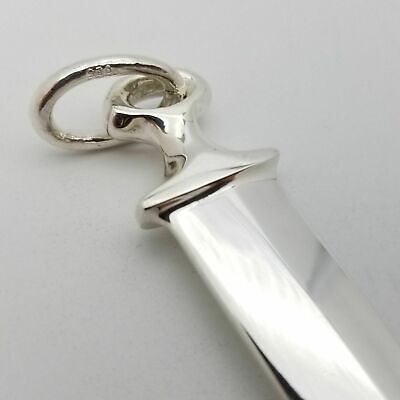The image showcases a close-up of a polished, shiny, metallic object against a plain white background. The central object appears to be the hilt or handle of a sword or perhaps a large knife, with a smooth, blade-like surface extending from it. This object has a loop or ring at one end that looks suitable for hanging, possibly on a wall rather than being carried by a person, suggesting it might be a decorative item or tool such as a letter opener. The ring itself has some kind of engraving, though the details are unreadable. The metallic surface of the object is reflective, with some subtle black shadowing and markings adding depth to the imagery. There is a noticeable raised line along the blade, adding texture to its sleek form.